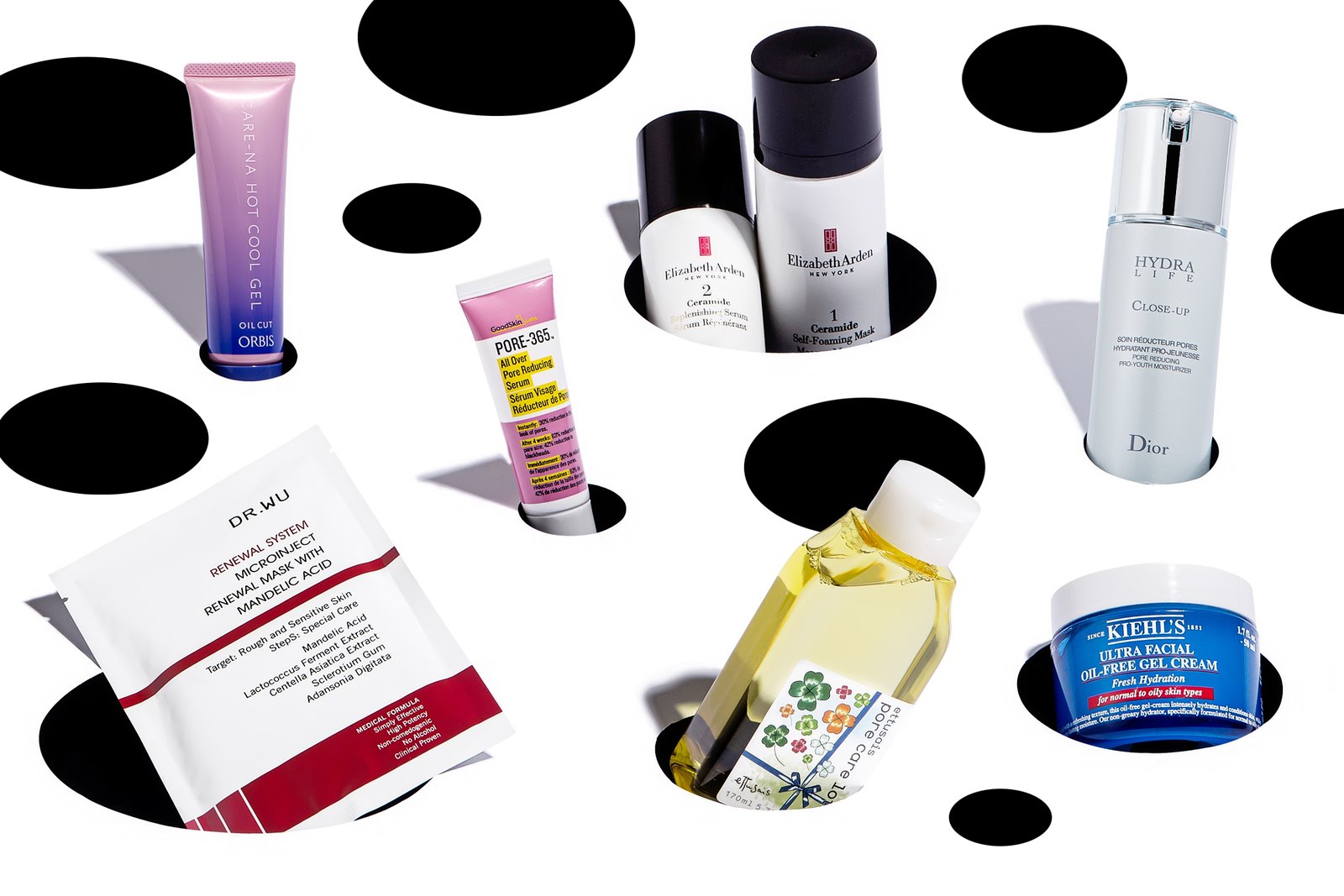The image displays a white surface dotted with small, black holes, each containing various skincare products. A total of eight products are showcased, including a face mask with white packaging and red bands, a bottle of micellar water with a white lid, and a small, blue container with a white lid labeled as an oil-free gel cream. Additionally, there is a tube with the word "PORE" prominently written on it, featuring a pink and white design with some text highlighted in yellow.